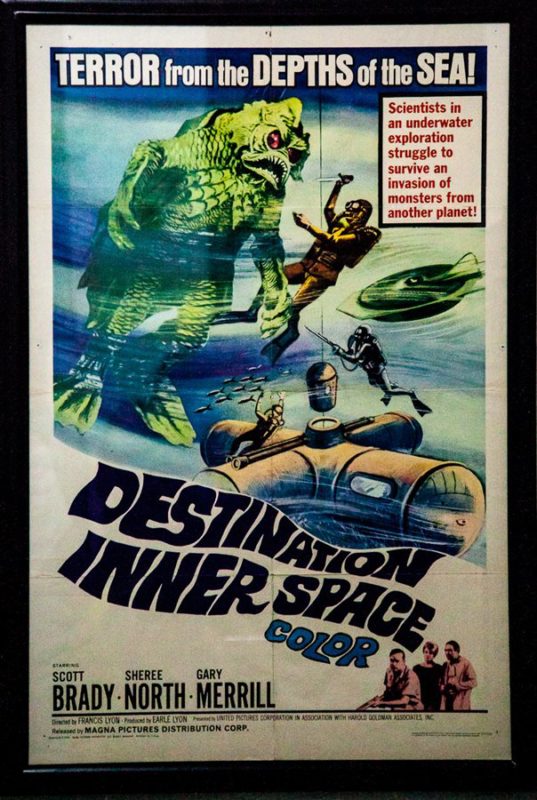This vintage movie poster, bordered by a black frame against a white background, vividly depicts the thrilling theme with the title "Terror from the Depths of the Sea!" in bold white letters atop a blue backdrop. Below, the tagline in red letters proclaims, "Scientists in an underwater exploration struggle to survive an invasion of monsters from another planet." The central image features a dramatic confrontation: a scuba diver armed with a knife fending off a vicious, green fish-like monster with legs and glaring eyes. Another diver is shown shooting at the creature, adding to the intense scene. The lower section of the poster showcases an underwater transportation device that resembles a cross-like submarine, surrounded by divers in full diving suits suggesting an underwater setting. The text at the bottom reads "Destination: Inner Space," and emphasizes that the film is in color. It stars Scott Brady, Cherie North, and Gary Merrill.